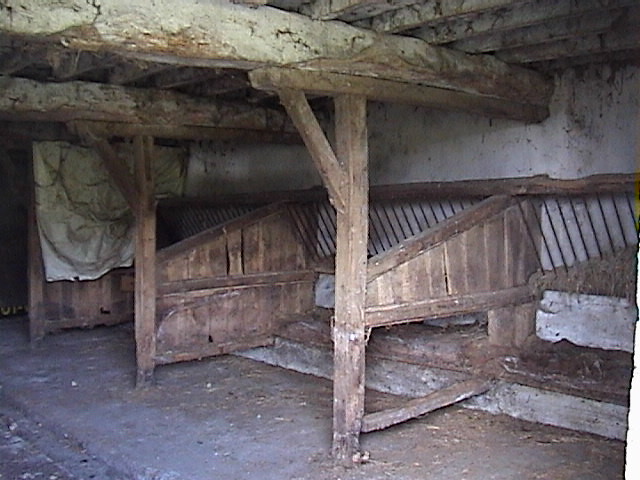The image captures a color photograph of a very rustic and dilapidated barn or old-style cellar. The floor appears dark, possibly concrete or dirt, contributing to the space's worn appearance. The concrete walls, particularly pronounced on the right side, extend into the background, merging with wooden sections that create stalls or divisions likely intended for horses or other livestock. Overhead, horizontal wooden roof trusses run parallel, supported by a much larger, thicker beam that stretches from the back right to the front left, emphasizing the rough, aged architecture.

The barn is cluttered with cobwebs, detritus, and decaying elements, enhancing its neglected look. Metal grates angled at 45 degrees are mounted on the back wall, with straw and hay visible through the bottom right grate, suggesting a functional design for feeding animals. Wooden posts, weathered and faded, support two main beams running left to right, with additional makeshift supports like a Y-shaped wooden brace. Along the back wall, wooden sections resemble a fence or shelf structure, interspersed with another wooden wall and draped with a dirty, white cloth. The overall scene evokes a sense of abandonment and disuse, with various elements blending together to paint a detailed picture of a profoundly aged and rustic space.